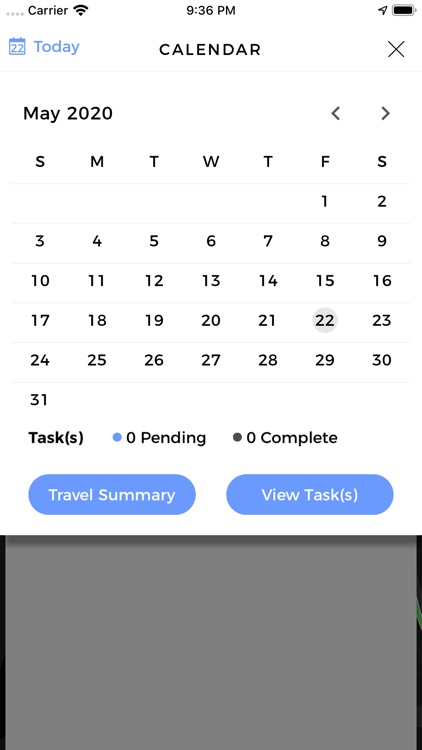The image depicts a screenshot of a digital calendar interface. At the very top left corner, the word "Carrier" is displayed alongside an emblem indicating an active internet connection. The time is shown as 9:36 PM, and there's a battery icon indicating the charge level.

Below "Carrier," the word "Today" appears prominently. A blue-colored date, "22," signifies the current day. Next to it, the word "Today" is printed, reinforcing the current date. To the right, the word "Calendar" is written, and further to the right, there's a large "X" symbol situated under the battery icon, possibly to close the calendar.

The period "May 2020" is prominently displayed in the left middle section of the interface. On the opposite side, there are left and right arrow icons allowing the user to navigate to previous or upcoming months.

Beneath this header, the days of the week are listed in abbreviated form: "S M T W T F S" for Sunday through Saturday. The first day of May begins on a Friday, and the month concludes on the 31st, which falls on a Sunday.

Further down, the section labeled "Tasks" is visible. In the middle are statistics indicating "0 pending" and "0 complete" tasks. There are two oval-shaped buttons labeled "Travel Summary" and "View Tasks."

At the bottom of the interface, there is an empty gray rectangular area outlined in black, possibly a space for additional information or interactive content.